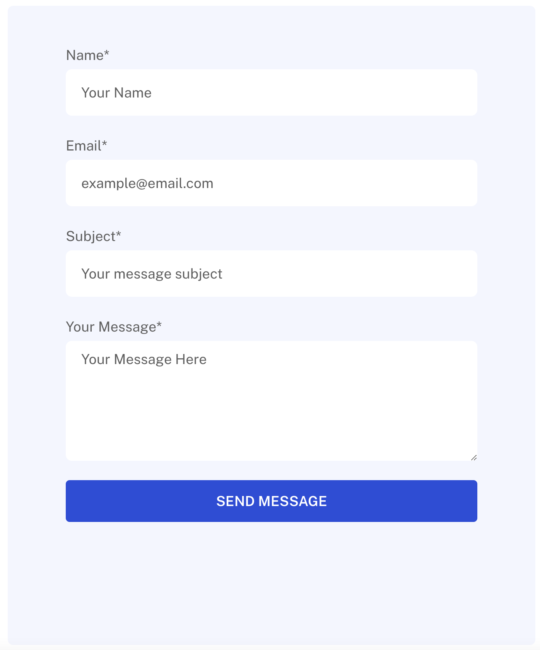The image features a very pale blue background. From the top, there is a black text that reads "Name" with a capital 'N'. Below this text, there is a white banner where "Your Name" is written, with both words capitalized (Y and N).

Further down, the text "Email*" appears, with the 'E' capitalized and an asterisk indicating a required field. Beneath this, there is another white banner containing the placeholder text "example@email.com".

Continuing down, the word "Subject*" is seen with a capital 'S' and an asterisk. Directly below this, there is a white space that holds the text "Your Message Subject", with each word starting with a capital letter (Y, M, and S).

Next, the text "Your Message*" appears, with 'Y' and 'M' capitalized and an asterisk, indicating another required field. Following this is a larger white space where "Your Message Here" is written in capitalized form for each word (Y, M, and H).

At the bottom of the image, there is a blue rectangular banner with a brighter blue interior. Inside this banner, the phrase "SEND A MESSAGE" is printed in white, capitalized text.